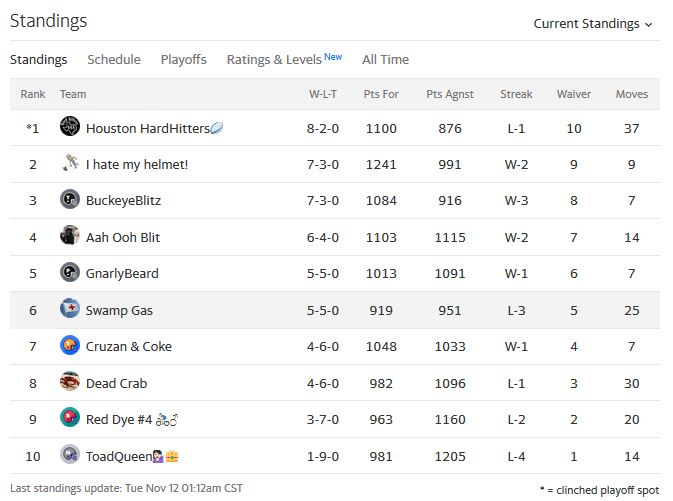Title: "Current Standings of the League"

Description: This detailed image displays the current standings of a league, prominently featuring a header titled "Standings." Below the header, a navigation bar allows users to switch between different categories, including "Standings," "Schedule," "Playoffs," "Ratings," and "Levels" (marked as "New"), as well as "All Time".

The standings list features ten teams, ranked from one to ten:

1. Houston Hard Hitters
2. I Hate My Helmet
3. Buckeye Blitz
4. Ah Ooh Blit
5. Gnarly Beard
6. Swamp Gas
7. Cruzan and Coke
8. Dead Crab
9. Red Dye
10. Toad Queen

Several team names are accompanied by emojis, adding a personalized touch. Each team is also represented by a small circle icon placed between their ranking number and name. 

Columns at the top of the standings provide detailed statistics for each team, including:

- WLT (Wins, Losses, Ties)
- Points For
- Points Against
- Streak
- Waiver
- Moves

This organized and comprehensive layout offers a clear and efficient way to track the performance and standing of each team in the league.